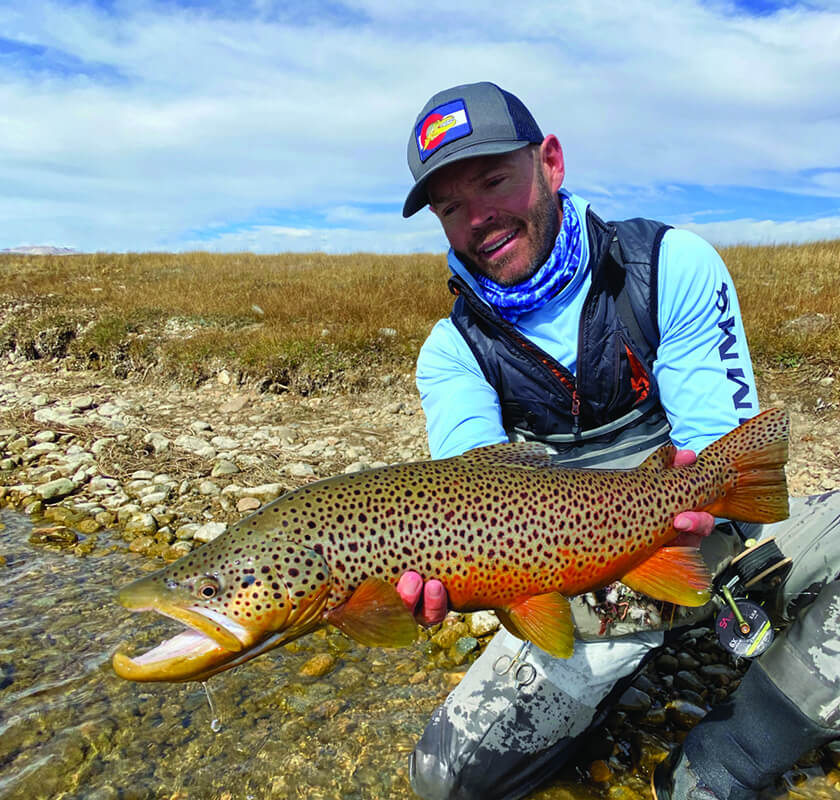In the image, a white man with a light brown beard is proudly kneeling in a rocky stream, showcasing a large fish he has caught. The man's attire is that of an avid fisherman: he dons a long-sleeved light blue "Sims" shirt, a gray vest, and brown and black fishing boot waders over white pants. A blue bandana is tied around his neck, and atop his head is a gray and blue Colorado trucker hat adorned with a red "C" and a yellow patch. The fish, held firmly in both of his hands, is striking with its massive, wide-open mouth that is ringed in a bright golden yellow. The fish's body is primarily green with scattered brown spots, and its underside and one of its fins exhibit a vibrant orange hue. In the background, a grassy field stretches out under a partly cloudy sky with some gray clouds and distant mountains visible to the left. The shore around the man is strewn with small boulders and rocks, indicative of a rugged outdoor setting perfect for fishing. The hook still hanging in the fish’s mouth suggests a fresh catch, making the display even more impressive.